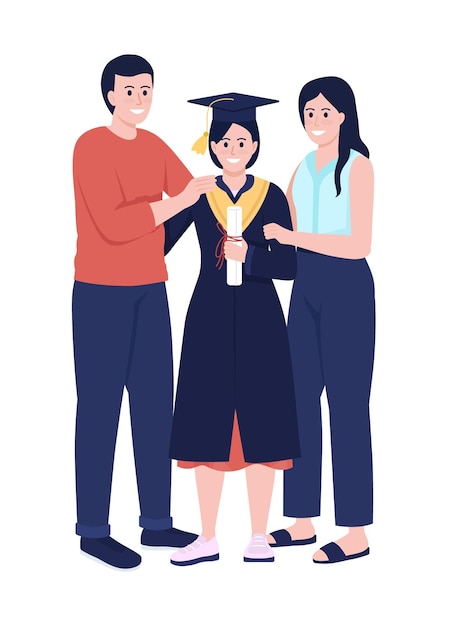This vividly colored and animated illustration features three cartoonish, celebratory figures against a white backdrop. The center of attention is a young woman celebrating her graduation, proudly wearing a black cap with a gold tassel, and a black graduation gown with a hint of yellow. Her short black hair frames a smiling face, and she holds a curled diploma tied with a red string. Beneath her gown, she dons a vibrant orange dress paired with pink shoes.

Flanking her on the left is a taller man, also beaming with pride. He wears a long-sleeved orange shirt, blue pants, and black shoes, with his right hand placed supportively on the graduate’s shoulder. To the right stands a woman with long black hair cascading past her shoulders. She sports a sleeveless blue top paired with blue pants and black open-toed sandals, with her left hand gently resting on the arm of the central figure. The rectangular image is twice as wide as it is tall, capturing a heartwarming family moment of achievement and joy.